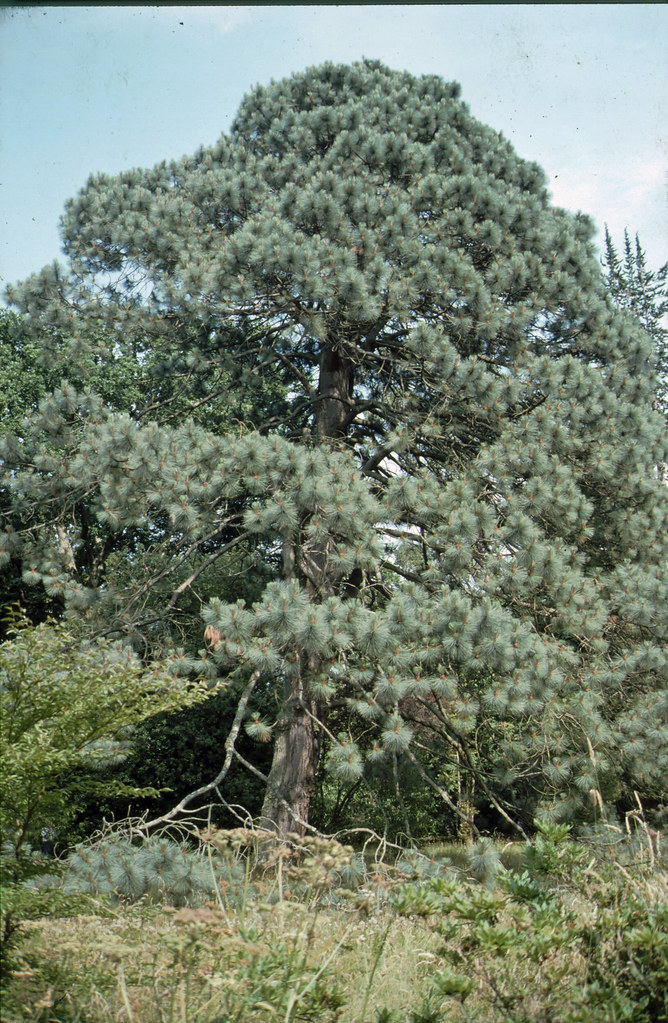This photograph captures a large, slightly tilting pine tree as its focal point. The tree, with its light green needles and a few barren branches, stands tall amongst surrounding greenery on a gently sloping terrain. To the left and right, different types of trees with varied foliage are visible, while the ground below features a mix of pine needles, weeds, and some grassy patches. The scene is set against a light blue sky with sparse clouds, indicating a bright and clear day. No human or animal presence is observed, and the background hints at human structures or a roadway subtly out of focus. The image, taller than it is wide, presents a serene snapshot of nature's quiet dominance.